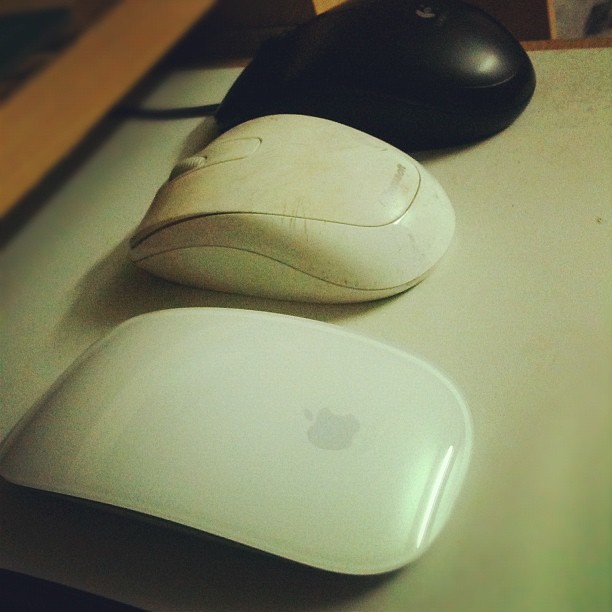This is a detailed close-up photograph of three computer mice arranged in a horizontal line on an off-white surface, likely a tabletop or desktop. The first mouse in the foreground is a sleek, glossy Apple mouse, clearly new and clean with the Apple logo visible. The second mouse is a well-used, dingy white mouse with a roller ball in the center, likely a Microsoft or Logitech model, showing signs of extensive use. The third mouse, positioned at the top of the photograph, is a black, glossy mouse with a visible cord running out of it, indicating it's wired, unlike the other two, which are presumably wireless. The mice are placed on what appears to be a whiteboard, with part of a brown frame visible along two sides, and a bit of shelving in the blurred background. The focus of the image is squarely on the three diverse and distinct mice lined up in an orderly fashion.